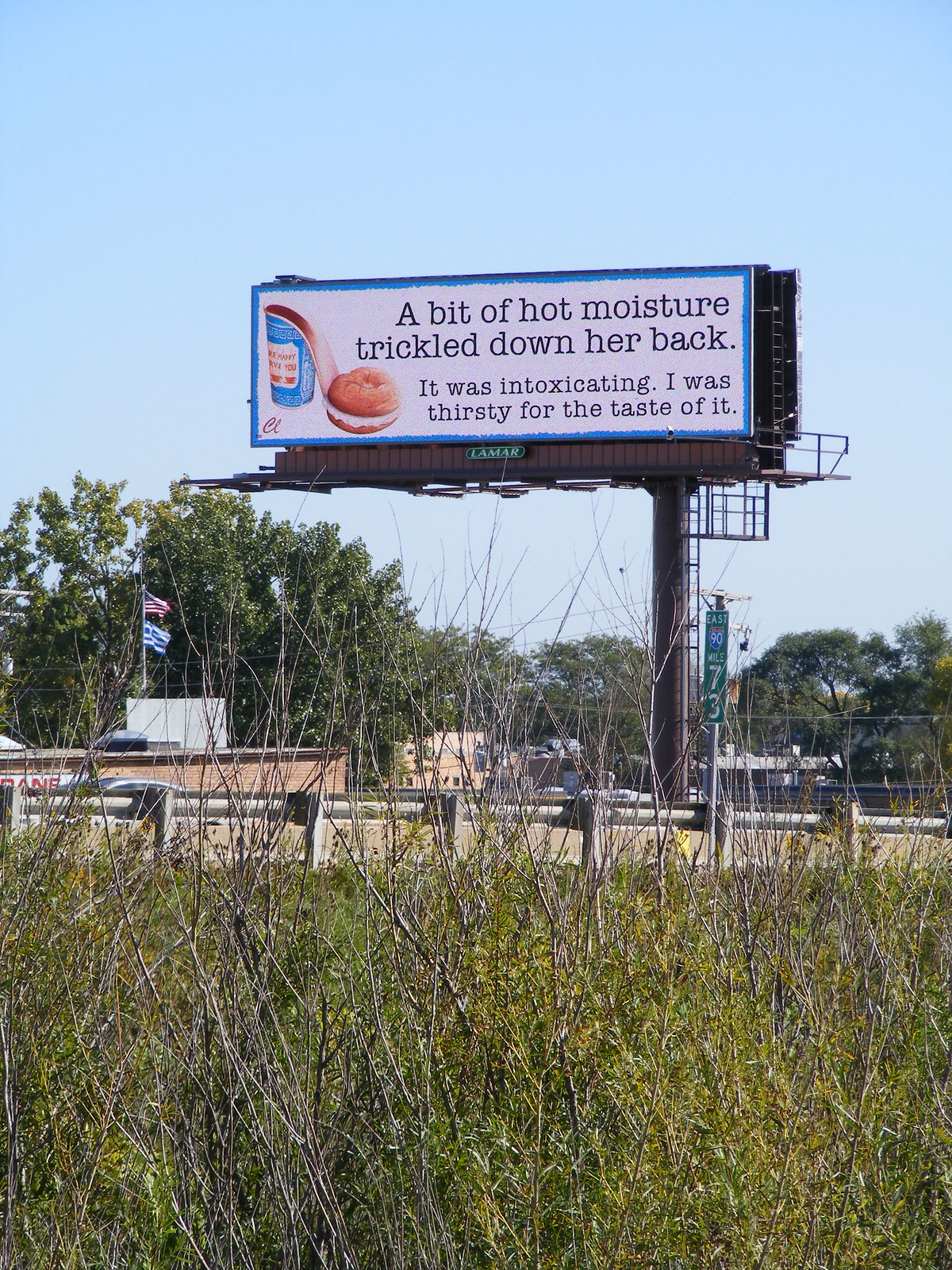This photograph captures a large, imposing billboard elevated on a substantial metal pillar equipped with a safety ladder along its side. The billboard stands prominently in an open expanse of long grasses and shrubs, showcasing a diverse palette of sage green, yellow-green, and dark green, interspersed with patches of dry twigs in brown and grey.

At the base of the billboard, there's an ambiguous structure that may be a raised pipeline or a low wall, beyond which a small building is visible. On the distant horizon, tall trees line the edge, gradually transitioning the sky from a pale blue near the horizon to a richer, starling egg blue higher up.

Among the trees, there's a building adorned with two flags, one prominently recognizable as an American flag.

The billboard itself consists of two panels angled to form a V-shape when viewed from above. It features a predominantly white face framed with a blue border. On the left side of the billboard, there's an indistinct object that might be a cup of coffee. Accompanying this image, the billboard bears a striking black text that reads: "A bit of hot moisture trickled down her back, it was intoxicating, I was thirsty for the taste of it."

The scene captures a sense of isolation and intrigue, juxtaposing the desolate, natural foreground with the stark, evocative advertising message on the billboard.